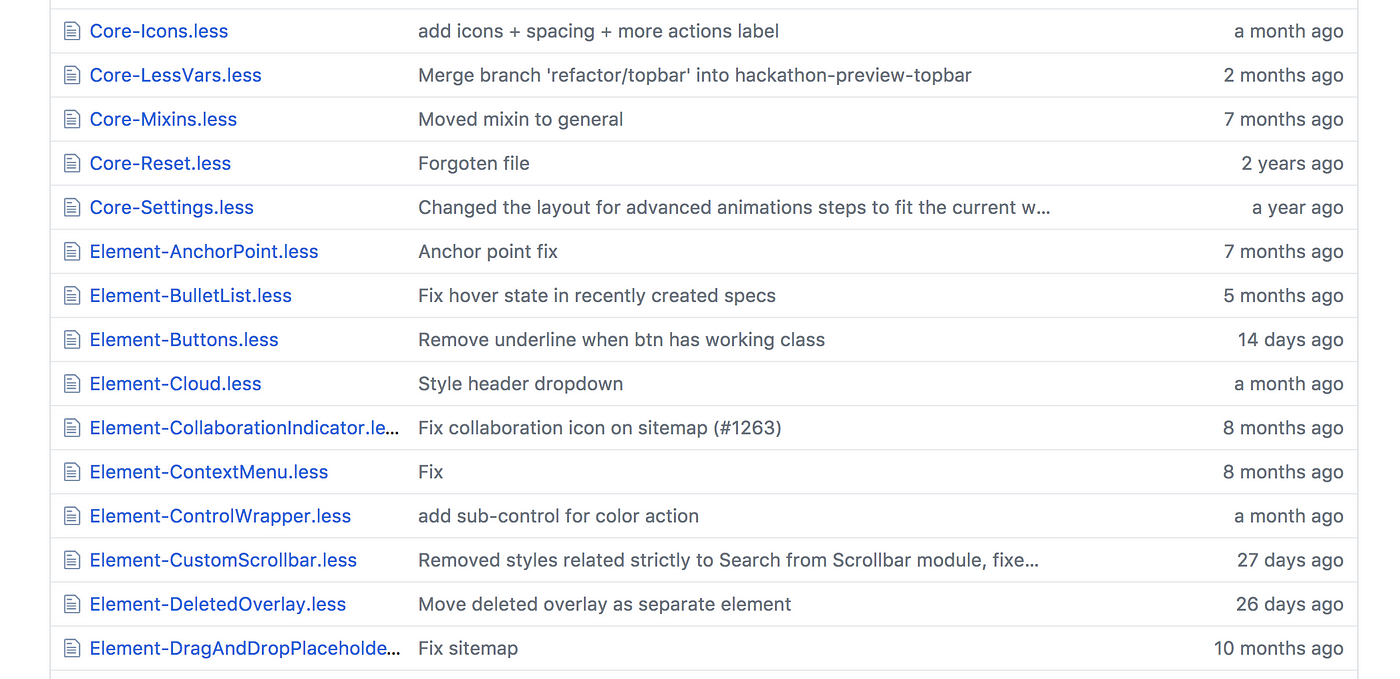This screenshot displays a detailed log of various updates and fixes made to a website or software application. The log is organized into three columns:

- The left column lists the filenames or document links.
- The middle column provides a description of the changes made.
- The right column indicates the timestamp of when each update was implemented.

Here are some specific entries from the screenshot:

1. **Left Column**: core-icons.less
   **Middle Column**: Add icons, spacing adjustments, and additional actions label.
   **Right Column**: A month ago

2. **Left Column**: core-dash-less-vars.less
   **Middle Column**: Merged branch 'refactor/top-bar' into 'hackathon-preview-top-bar.'
   **Right Column**: Two days ago